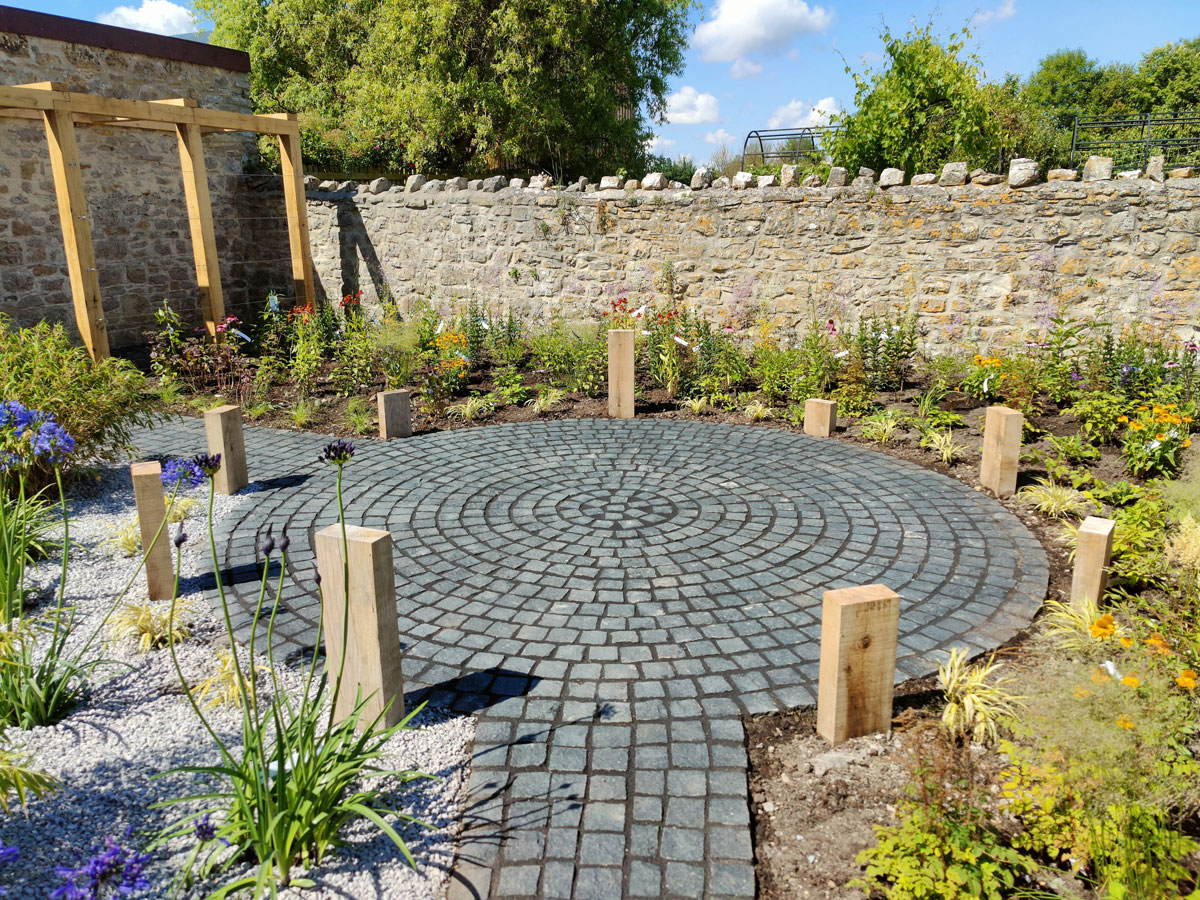The image depicts a lush outdoor garden scene under a bright blue sky dotted with a few white clouds. Dominating the center is a circular area paved with various gray concrete or stone tiles, surrounded by wooden blocks of different sizes embedded in the ground. Leading up to this circle is a pathway also lined with tiles, which extends to the left. On the left side of the image, there's a newly built wooden frame or trellis, suggesting ongoing construction. The garden is bordered by a taller gray stone wall, topped with individual stones, and is adorned with a variety of plants, shrubs, flowers, and some weeds. In the distance, additional greenery and trees add depth to the scene. The backdrop features a robust stone wall, further enhancing the rustic and serene atmosphere of this garden.